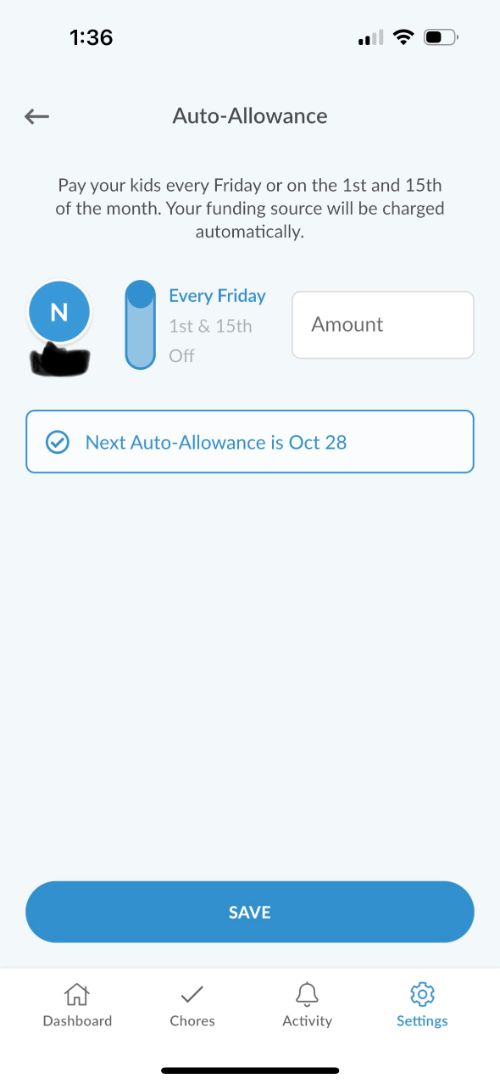**Detailed Caption:**

This screenshot captures a section of a parenting app in light mode, specifically the "Auto Dash Allowance" feature. The current time displayed is 1:36 PM. This section offers parents the option to pay their kids' allowances automatically on various schedules: every Friday, the first and 15th of the month, or to turn off the auto payment altogether. The selected option here is "Every Friday." The app indicates that your funding source will be charged automatically.

Towards the right, there's a text field intended for the amount to be paid, which is currently blank. Below the scheduling options, there is a message stating "Next auto allowance is October 28th," written in blue text on a white background, accompanied by a checkmark to the left of the message.

At the bottom of the section, a prominent blue "Save" button is visible, allowing users to save their settings. Additional tabs are present at the bottom of the screen, specifically "Dashboard," "Chores," "Activity," and "Settings," with "Settings" currently active. The screenshot appears to be taken from an iOS device, utilizing the light mode interface. Some user-related information is blurred out next to an "N" icon, suggesting the app personalizes the experience for different users.